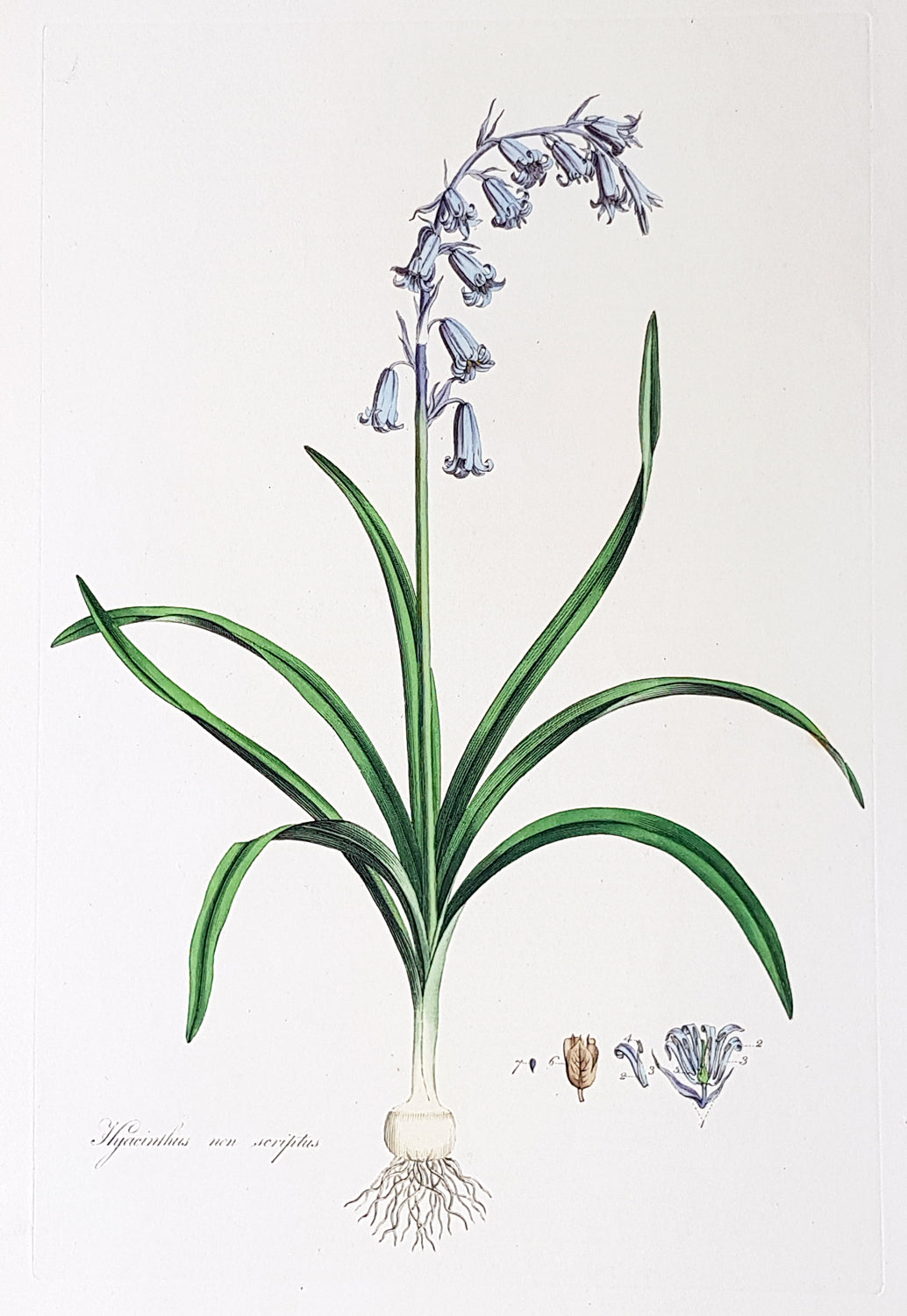This detailed illustration depicts a flowering plant with a distinctive violet and bluish hue. The main focus is on the large central flower, which appears to be composed of numerous smaller blossoms merging together. Positioned at the base of the plant is a bulbous structure resembling an onion, with multiple roots extending downward into an implied, though invisible, soil. The background is a light, neutral blend of white and beige tones.

On the right side of the image, there is a diagrammatic sequence illustrating the plant's blooming process, starting from a small seed at the lower right corner. This seed progresses into a brown, cupped pre-blossom stage before evolving into a small purple-violet flower. This flower multiplies, eventually forming the larger, composite flower depicted in the center.

The plant's green leaves, which initially droop downward like those of a spider plant, curve upward as they ascend the stem. The flowering stem is adorned with approximately 11 or 12 undeveloped bulbs that are violet with a hint of blue. Some of these bulbs also have leaves tinged with purple and violet. 

In the bottom left corner of the painting, there is a barely legible, light gray signature, presumably of the artist. While the exact plant species is uncertain, it shares characteristics with hostas or bluebells. The overall color palette includes light gray, green, violet, blue, and white, contributing to the harmonious appearance of the image.